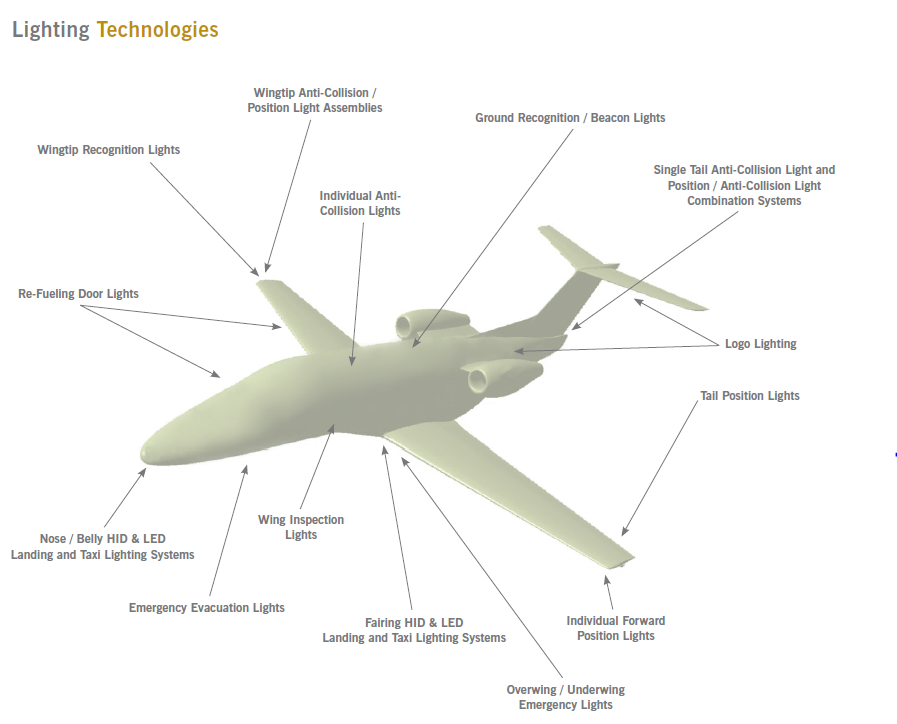The image is a detailed diagram on a white background, depicting various lighting technologies on a Learjet airplane. There is no border around the image. In the upper left-hand corner, it reads "Lighting Technologies," with "Lighting" in gray and "Technologies" in tan. Central to the diagram is a computer-generated, off-white outline of a Learjet, depicted without any windows, cockpit details, or airline logos.

The diagram is annotated with multiple black-lettered labels, each connected by gray arrows pointing to specific parts of the plane. Starting from the top-left and moving clockwise, the labels identify various lighting components: "Wingtip Recognition Lights" and "Wingtip Anti-Collision/Position Light Assemblies" pointing to the wings; "Logo Lighting" pointing to the tail; "Refueling Door Lights" pointing to a section on the wing and front end.

Additionally, other annotations include: "Individual Anti-Collision Lights," "Ground Recognition/Beacon Lights," "Single Tail Anti-Collision Light and Position Light Combinations," "Tail Position Lights," "Individual Forward Positioning Lights," "Overwing/Underwing Emergency Lights," "Fairing HID and LED Landing and Taxi Lighting Systems," "Wing Inspection Lights," "Emergency Evacuation Lights," and "Nose/Belly HID and LED Landing and Taxi Lighting Systems." The diagram is densely populated with text and arrows thoroughly mapping out the various lighting systems employed on the aircraft.